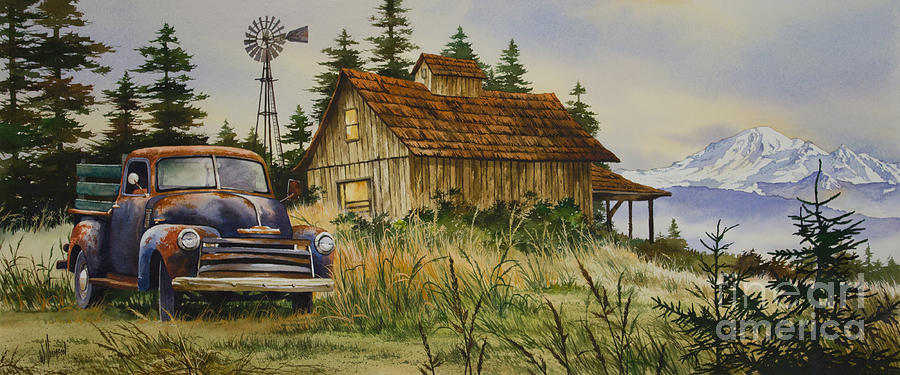In this evocative painting, a rustic wooden farmhouse, distinguished by its brown color and triangular roof, stands amidst lush grassy ground. The farmhouse, centrally located, features a window and a door, with a warm, inviting light glowing inside. To its left, there's an old, blue truck, a relic of the 1940s, with significant rust on its fenders and roof, adding to the nostalgic charm of the scene. Behind the house, a tall windmill towers over, accompanied by a cluster of trees, possibly oak or pine. Beyond them, majestic mountains with snowy peaks rise in the background, extending from the right side of the frame. Above, the sky transitions from blue to cream, enhancing the serene atmosphere. In the bottom right corner, a faint watermark reads "Fine Art America," hinting at the painting's likely origin. This idyllic depiction, possibly set in the Midwest, invokes a simpler, pastoral lifestyle of the past.